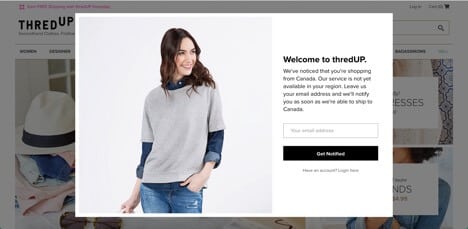The image depicts a user interface from the ThredUp website, with the logo "ThredUp" prominently displayed, where "UP" is shifted up half a line. The interface showcases various photographs of women's clothing, including sunglasses, a hat, and neatly folded T-shirts. On the right side, there is a partially visible woman with curly brown hair, wearing a light blue shirt, behind a white text field.

Dominating the center of the screen is a white pop-up window, obscuring most of the background content. The pop-up features a Caucasian woman with brown, wavy hair that falls just past her shoulders. She is wearing jeans, a long-sleeve button-down shirt with partially rolled-up sleeves, and a gray T-shirt layered on top. Her left hand is casually tucked into her front jean pocket, and she is smiling at the camera while slightly turning towards the right side of the screen.

On the right side of the pop-up, bold text reads, "Welcome to ThredUp." Below this, there is a notice indicating the user is shopping from Canada, followed by an input field. The pop-up also includes a black button with text that is difficult to discern, possibly saying "Get Started" or something similar, with more unreadable text below it. The rest of the interface has a semi-transparent black overlay, giving the background a screened effect, estimated at 30 to 40% opacity.